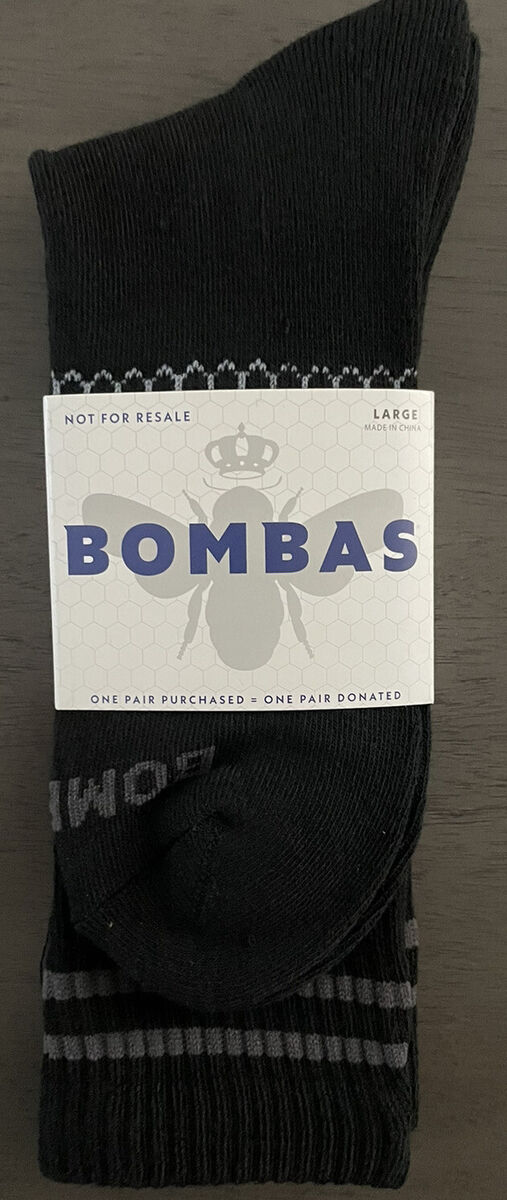This is a detailed photograph of a pair of black Bombas socks, presented in a vertical rectangular format against a dark gray background. The socks are neatly folded, occupying almost the entire height of the image, with the top portions positioned toward the bottom. The socks feature gray horizontal stripes near the top, as well as gray stitching around the foot area. They're still wrapped in white packaging that spans the middle section. The packaging prominently displays the Bombas logo in large blue font, accompanied by an illustration of a crowned bee. Additional text on the packaging includes "not for resale," "large," "made in China," and "one pair purchased equals one pair donated." Below this main label, you can faintly make out the partial text "B-O-M" on the foot part, hinting at the full Bombas branding. The socks rest on a table that appears to be a grayish-brown faux wood surface, although the image is closely cropped, focusing primarily on the socks.